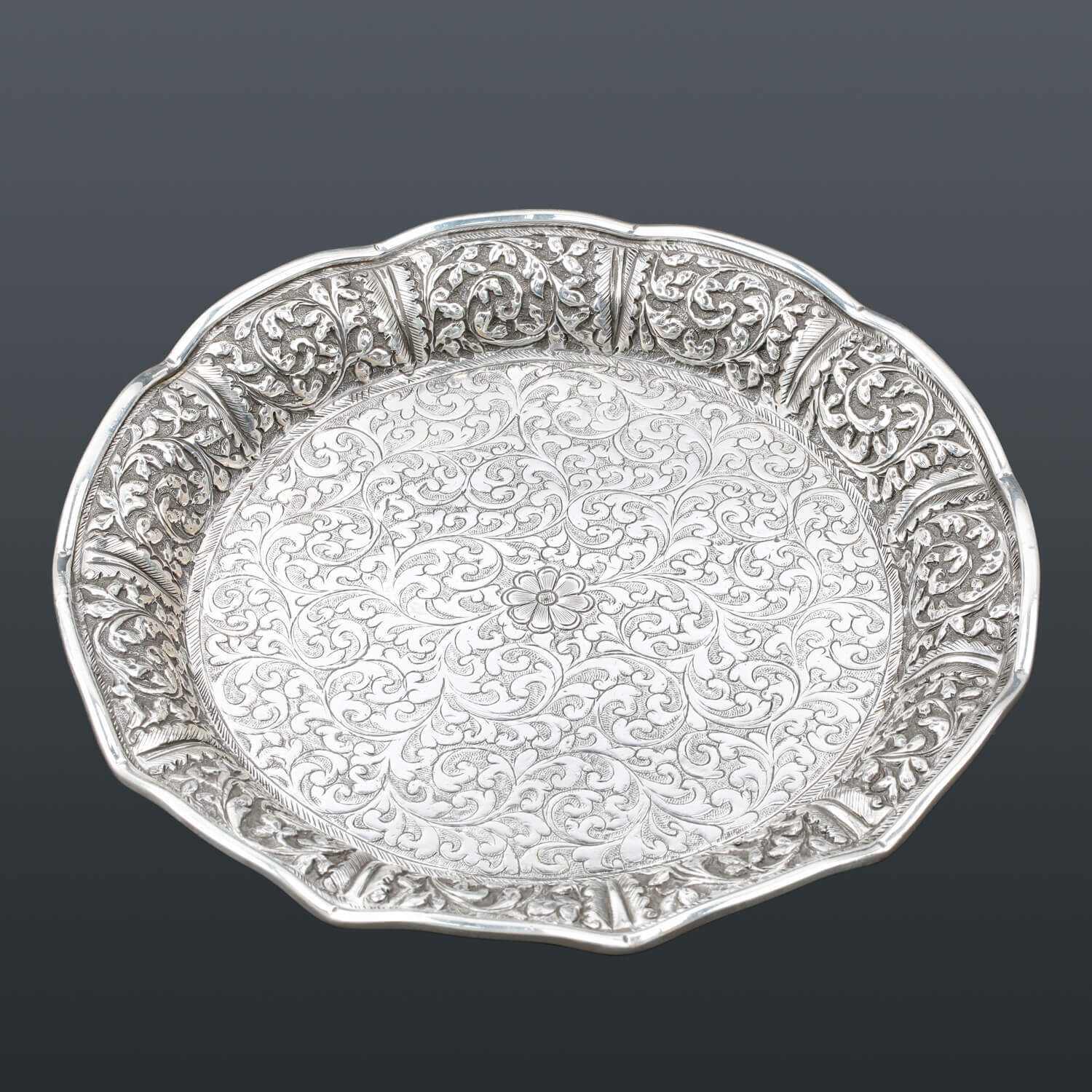This photograph captures a beautiful, vintage, silver or pewter plate, centered against a dark gray background. The plate features a detailed floral pattern, accented with silver, that adorns its scalloped, flanged rims. The central area of the plate showcases a prominent flower design, with intricate floral motifs extending around the entire bottom and sides. The plate's color palette consists of dark gray, light gray, and white. The plate appears old, displaying a subtle patina that adds to its charm, while it remains clean and visually striking. The background is darker at the top of the image, emphasizing the plate's centered positioning. The overall aesthetic suggests it could be an antique, possibly Victorian, poised as if showcased for an auction or displayed as part of a personal collection.